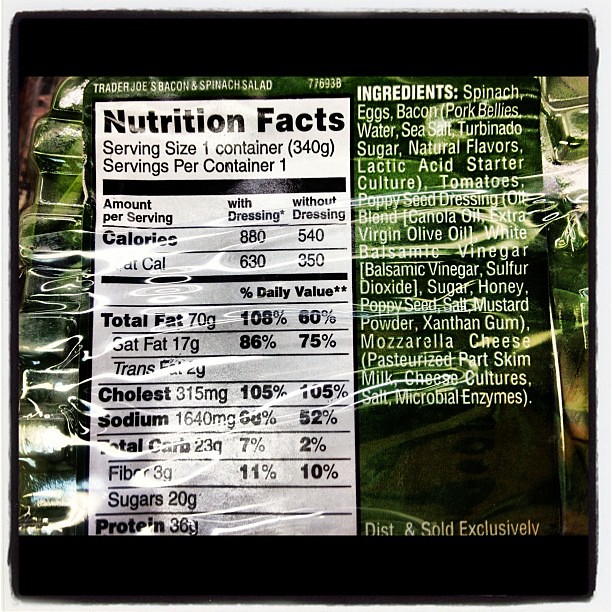This image is a color photograph depicting the back of a food package for Trader Joe's Bacon and Spinach Salad. The packaging features a green background, with nutritional information prominently displayed in a white rectangle outlined in black at the center. At the top left of the packaging, "Trader Joe's Bacon and Spinach Salad" is printed in white text. The nutrition facts state that the serving size is one container, which is 340 grams, with one serving per container. The salad contains 880 calories with dressing and 540 calories without dressing. It has 70 grams of total fat, including 17 grams of saturated fat and 2 grams of trans fat. The cholesterol level is listed at 105% of the daily value, and sodium is at 68%. The nutritional breakdown continues with total carbohydrates being 23 grams, 20 grams of sugar, and 6 grams of protein. Detailed percentages for daily values are also provided for various nutrients.

The ingredients, written in white over the green section, include spinach, eggs, bacon (pork bellies, water, sea salt, tomato, sugar, natural flavors, lactic acid, starter culture), tomatoes, poppy seed dressing (canola oil blend, extra virgin olive oil, white balsamic vinegar, balsamic vinegar, sulfur dioxide, sugar, honey, poppy seed, salt, mustard powder, xanthan gum), mozzarella cheese (pasteurized part-skim milk, cheese culture, salt, microbial enzymes). The bottom right corner indicates the salad is "distributed and sold exclusively" at Trader Joe's. Additionally, there are black rectangles above and below the nutritional information, and some green produce is visible behind the plastic packaging.